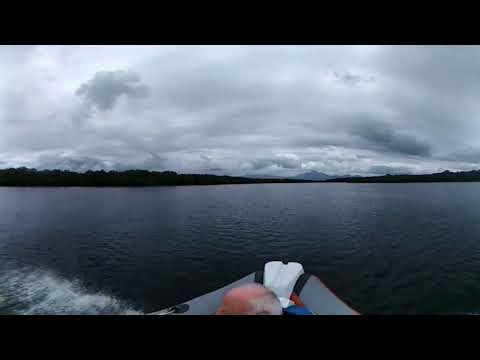The image depicts a tranquil scene of calm, dark gray water that encompasses the lower half of the frame, punctuated by gentle waves emanating from a vessel. In the foreground center, the bow of a boat or raft, painted in blue with accents of white and black, commands attention. A lone figure aboard the vessel catches the eye: a man with a bald, partially gray-haired head turned slightly to the side, obscuring detailed facial features. The horizon is marked by a thin, undulating black line of distant trees, which gives way to a serene landscape featuring a mountain in the far center background. Above, the sky is heavy with white and gray clouds, lending a wintry, subdued atmosphere to the scene. The absence of other boats, wildlife, skiers, or swimmers underscores the solitary calmness of what appears to be a lake, framed by the untouched natural beauty of its surroundings.